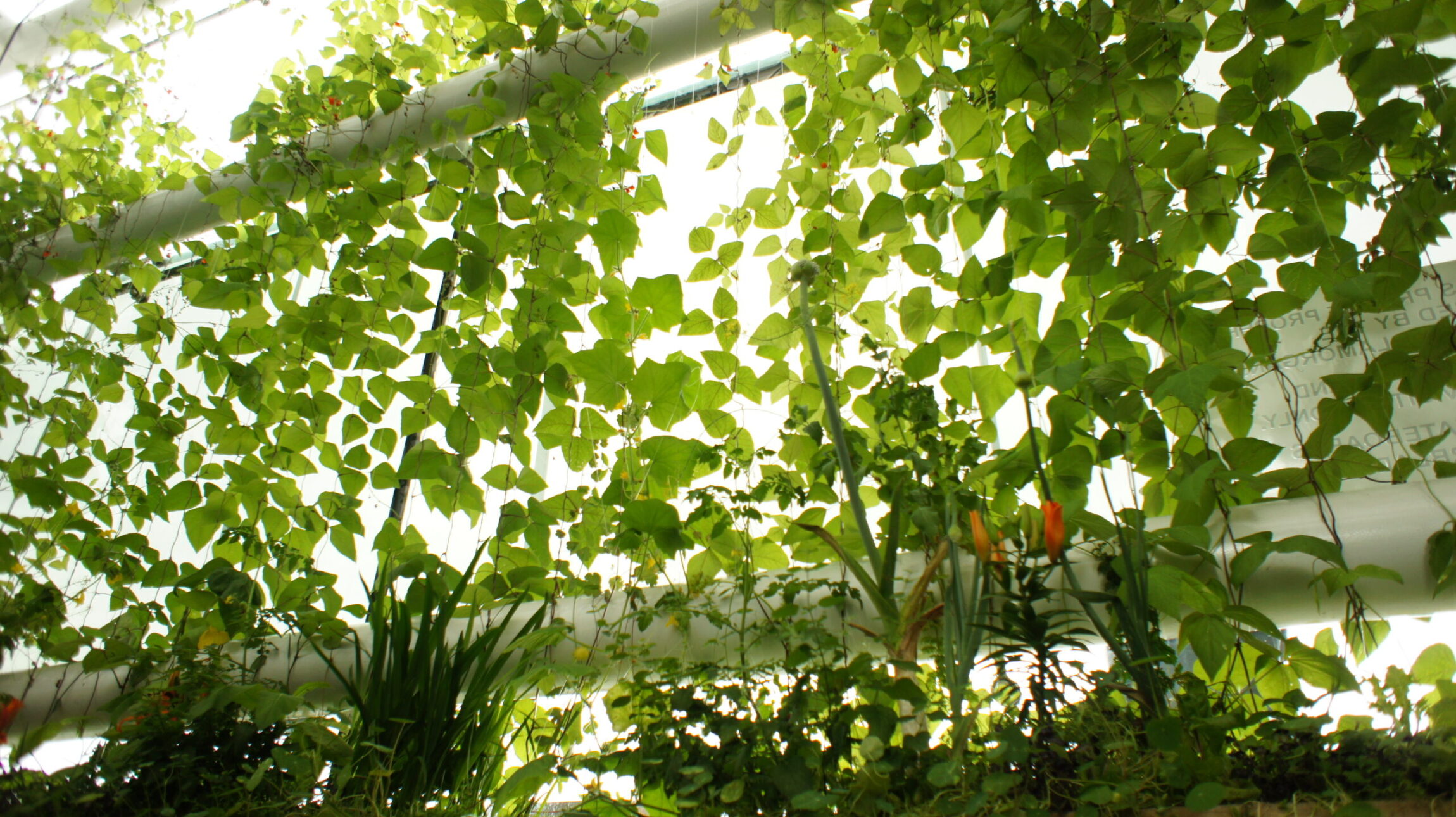This color photograph, taken outdoors, showcases an array of hanging vines suspended from two long white PVC pipes, one at the top and another near the bottom of the image. The vines stretch down gracefully, their greenery capturing the sunlight that filters through gaps in the leaves. In the foreground, various smaller plants and shrubs are visible, featuring slender blade-like leaves and distinctive orange and yellow flowers, likely lilies in the process of blooming. Adding to the scene's vibrant diversity are two small red flowers that stand out among the foliage. On the far right side, partially obscured by the plants, is a red sign seen from the back, its writing not legible. The composition is devoid of people, focusing entirely on the thriving, sunlit plant life.